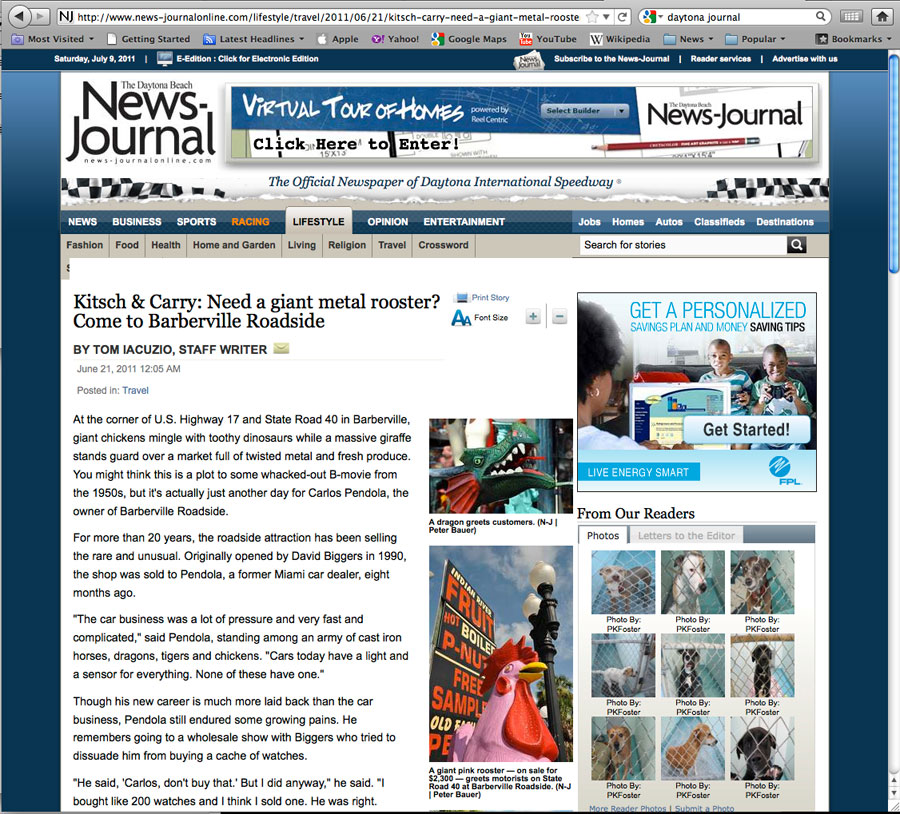The screenshot exhibits a webpage of the Daytona Beach News Journal’s e-edition, dated Saturday, July 8th, 2011. The webpage is accessed from a computer, evident by the interface elements such as a search bar at the top, most visited sites, and bookmarks. A darker blue bar prominently displays the date in white text and marks it as the Daytona Beach News Journal. The publication’s name is shown in varying font sizes; "Daytona Beach" appears smaller and in light gray, while "News Journal" is significantly larger.

To the right, there is a clickable link offering a virtual tour of homes, indicating a contest entry. Below this, the page is organized into various sections including News, Business, Sports, Racing (in orange), Lifestyle, Opinion, Entertainment, and further right categories such as Jobs, Homes, Autos, Classifieds, and Destinations. The section currently highlighted is "Lifestyle," denoted by a gray background.

Beneath this, there is a mention of "Personalized Savings Plan" from readers, followed by different images featuring dogs from pounds. A highlighted article titled "Kitchen carry: Need a giant metal rooster? Come to Barbosville" appears, penned by staff writer Tom on June 21st. The article discusses a unique kitchen item alongside two accompanying images: one of a dragon greeting a customer and a pink rooster priced at $2300.